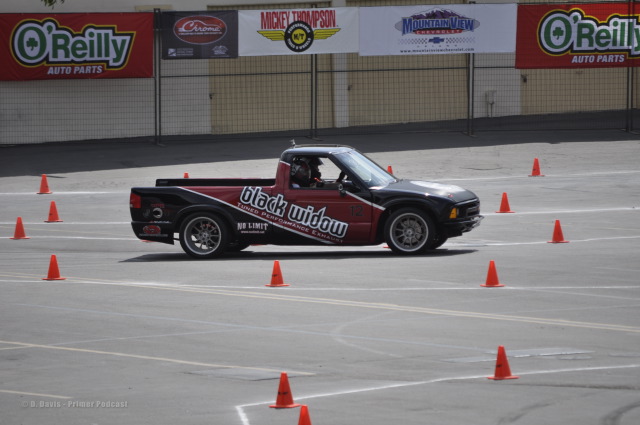The image depicts a small black pickup truck with a red diagonal stripe and the words "Black Widow" emblazoned in black letters with white outlines across the hood. The truck, which has silver-rimmed tires, is situated in the center of a gray paved lot and faces to the right. It is positioned among numerous orange traffic cones, suggesting it is navigating a driving course. The lot is outlined with white lines, adding to the structured appearance of the course. A driver is visible behind the wheel of the truck. 

In the background, a chain-link fence adorned with several advertising banners separates the lot from the surrounding area. The visible banners include two for O'Reilly Auto Parts, one on the far left and one on the right. Other banners promote brands like Mickey Thompson and Mountain View, as well as another banner that says "Krim." Behind the fence, a white building with beige garage doors can be seen, further situating the scene within a racetrack or event space environment.